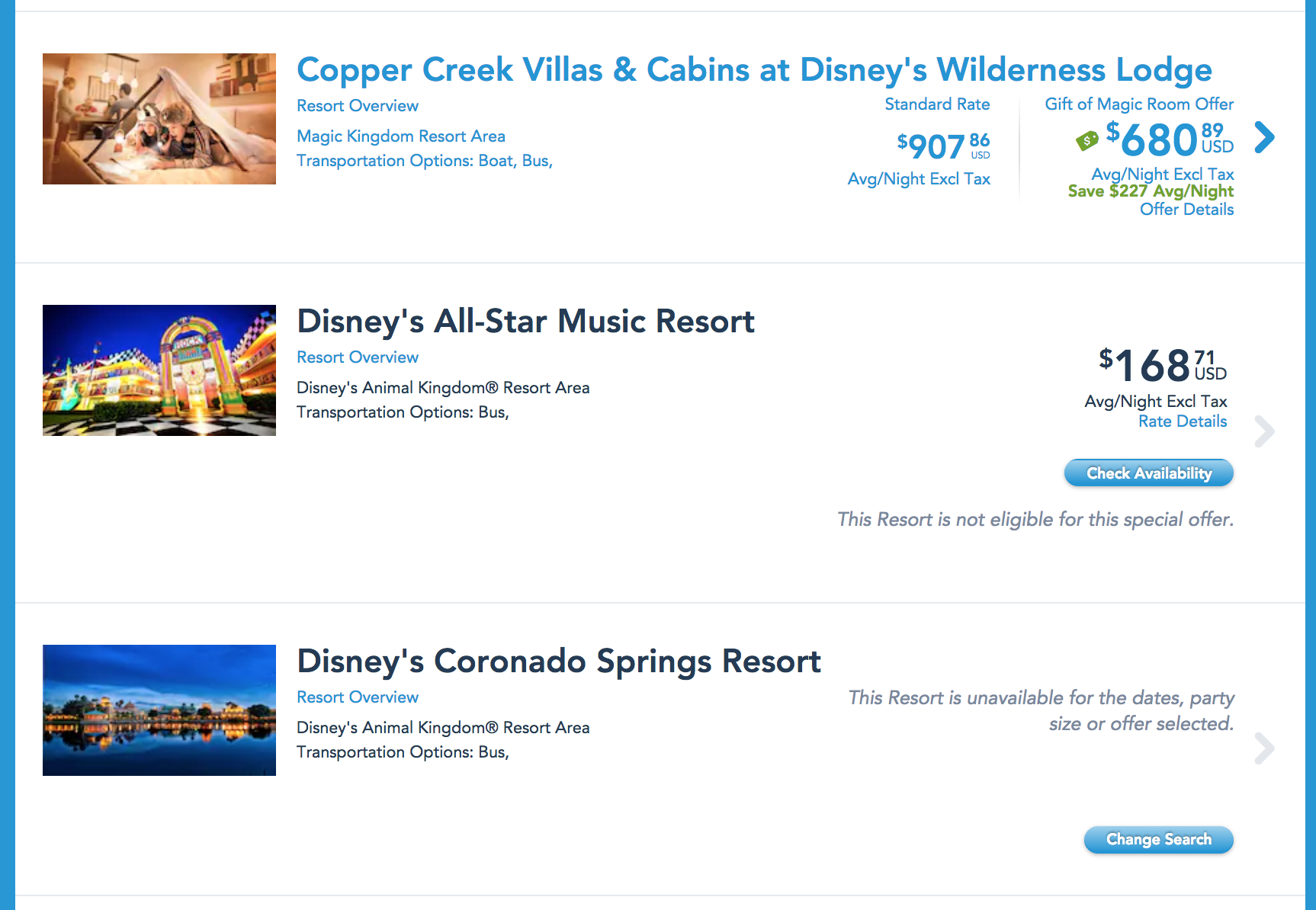This screenshot features a travel website interface, likely related to Disney resorts, but devoid of any definitive branding. The layout displays blue bars on either side of the screen. In the top-left corner, there is an image depicting two children building a fort on a bed, with people visible in the background near a dining table.

Highlighted in blue text, several resort options are listed with detailed information:

1. **Copper Creek Villas & Cabins at Disney’s Wilderness Lodge**
   - Overview: Located in the Magic Kingdom Resort area.
   - Transportation: Bus service available.
   - Standard Rate: $907.80 per night (excluding taxes).
   - Special Offer: Gift of the Magic Room for $680.89 per night (excluding taxes), saving $226 per night.
   - Offer Details & Availability: Additional information provided but not detailed in the caption.

2. **Disney’s All-Star Music Resort**
   - Overview: Situated in Disney’s Animal Kingdom Resort area.
   - Visual: A night-time shot featuring neon signs and what appears to be a jukebox.
   - Transportation: Bus service available.
   - Standard Rate: $160.71 per night.
   - Special Offer: This resort is not eligible for the mentioned special offer.
   - Availability Options: Information on how to check availability.

3. **Disney’s Coronado Springs Resort**
   - Overview: Located within Disney’s Animal Kingdom Resort area.
   - Visual: A hotel building is beautifully reflected in a lake.
   - Transportation: Bus service available.
   - Availability: This resort is currently unavailable for the selected dates or party size; however, there’s an option to change the search criteria.

Overall, the page appears to present options for booking stays at various Disney resorts, detailing nightly rates, available offers, and transport options. It remains ambiguous whether the site is a general travel agency platform or an official Disney site.